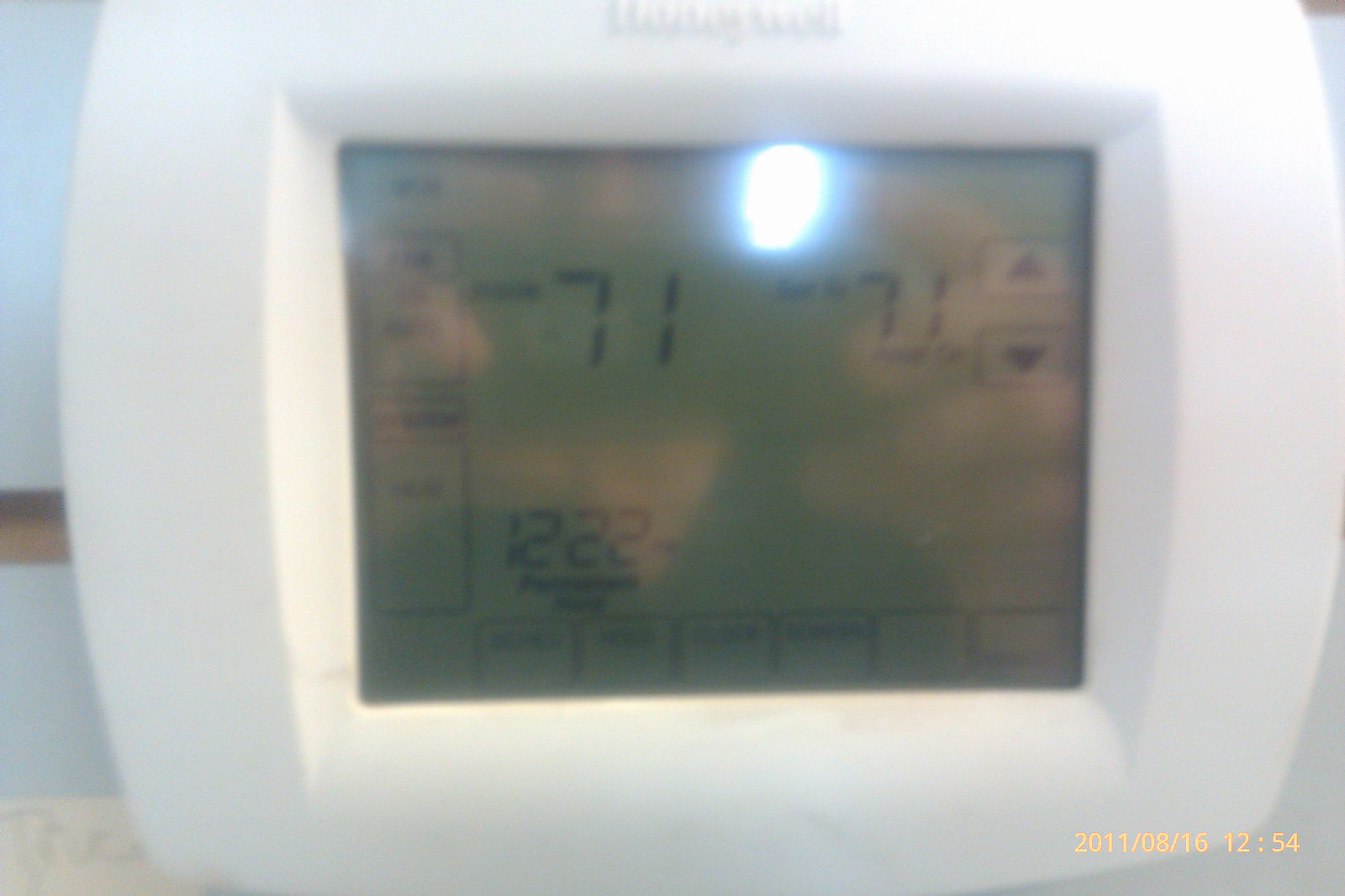The image depicts a digital dashboard interface with a white border. At the top-center, the word "honey" is prominently displayed. Beneath it, a light emanates from the top section of the screen, creating a subtle glow. The display background has a gradient of light yellowish-green to tan. The screen prominently shows the number "71."

To the right, there is a pair of buttons for navigating up and down. Below these buttons, the number "1222" is displayed. The interface features additional interactive buttons arranged around the perimeter.

In the bottom-right corner, the timestamp "2011/08/16 12:54" is written in a light orange hue, providing a precise date and time.